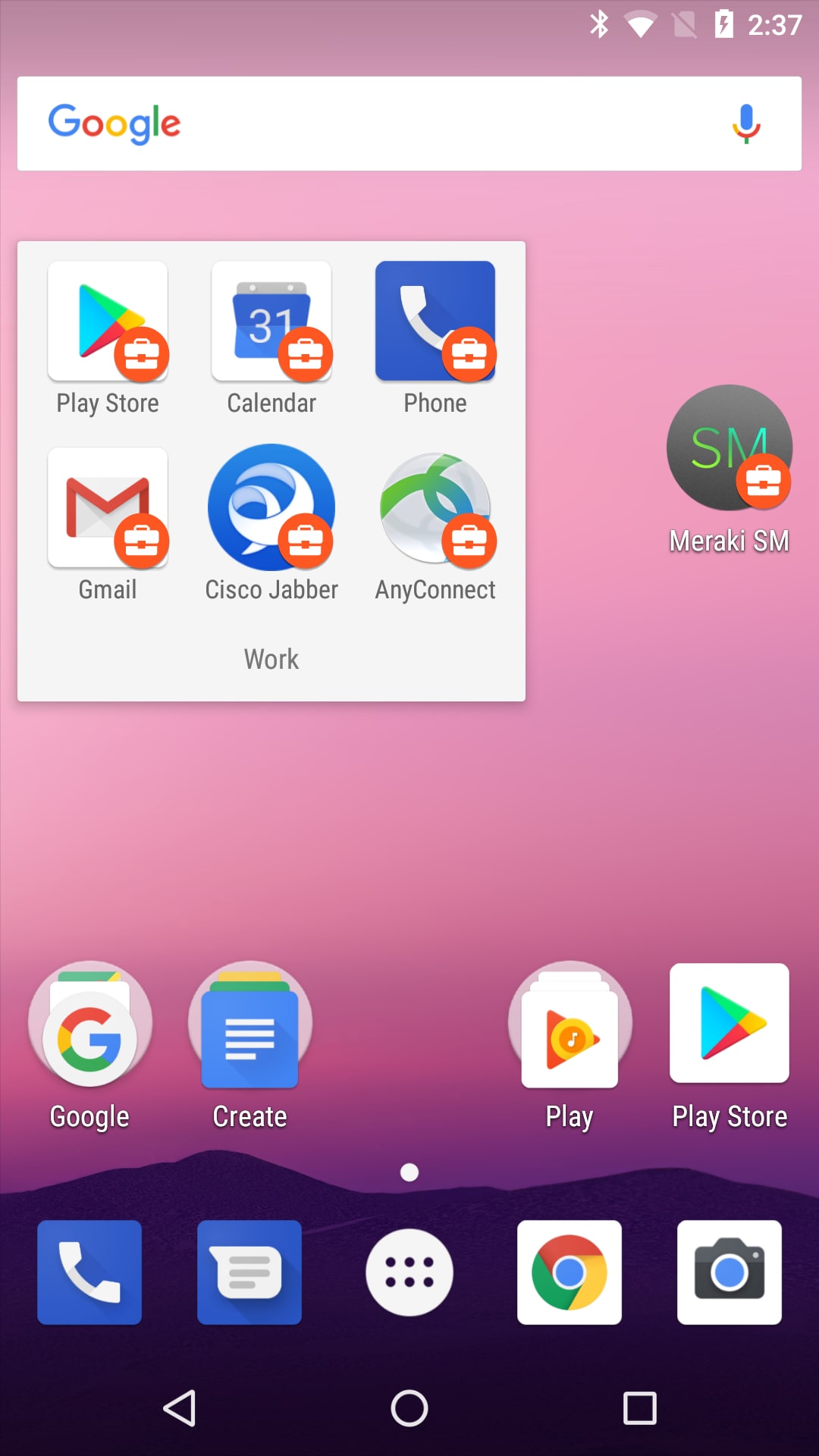The image is a vertically rectangular screenshot taken from a cell phone display. At the top left corner, the status bar displays icons for Bluetooth, Wi-Fi, and battery, next to the current time, 2:37. Below the status bar is a horizontal white banner featuring the Google logo on the left, a search text area in the center, and a microphone icon on the right.

Centered below this banner is a white background box labeled "Work" at the bottom. Inside this box are six app icons: Play Store, Calendar, Phone, Gmail, Cisco Jabber, and AnyConnect. To the right of this box is a circular icon labeled "SM" with "Meraki SM" written beneath it.

At the bottom of the image, there are two rows of icons. The top row consists of Google, Create, Play, and Play Store. The bottom row features icons for Phone, Text, the Menu button, Chrome, and Camera.